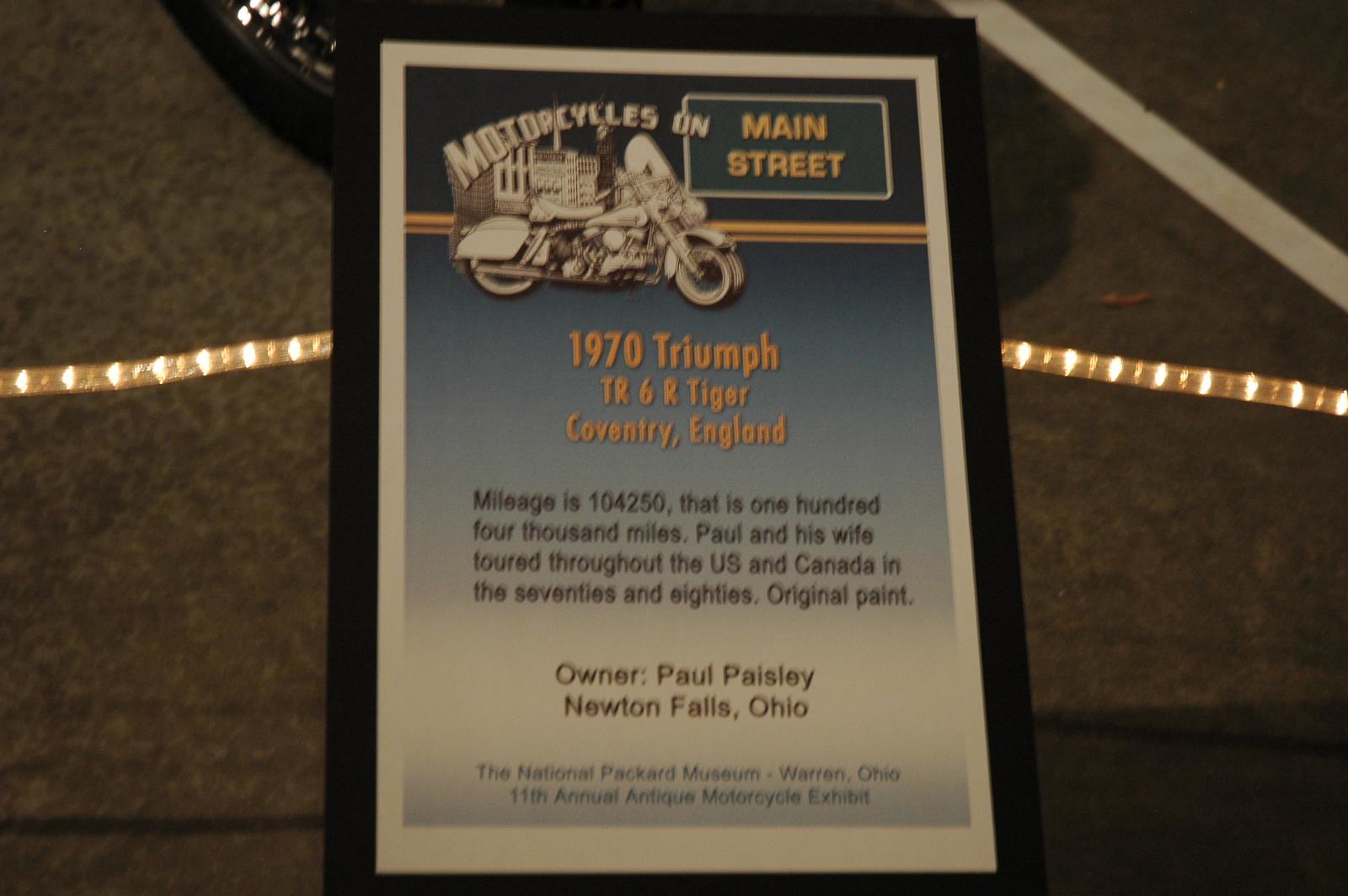This is a photograph of a poster propped against a backdrop of amber string lights, possibly taken at night in a parking lot. The pavement below shows a gray surface with a white parking line and a black vehicle parked nearby. The poster itself appears focused on a motorcycle display, titled "Motorcycles on Main Street", with a vintage motorcycle illustration at the top. It details a 1970 Triumph TR6R Tiger from Coventry, England, stating it has 104,250 miles. The story describes Paul and his wife's tours throughout the U.S. and Canada during the 70s and 80s, and highlights that the motorcycle retains its original paint. The owner is listed as Paul Paisley from Newton Falls, Ohio. Additionally, in smaller blue print, it mentions the National Packard Museum's 11th Annual Antique Motorcycle Exhibit in Warren, Ohio.